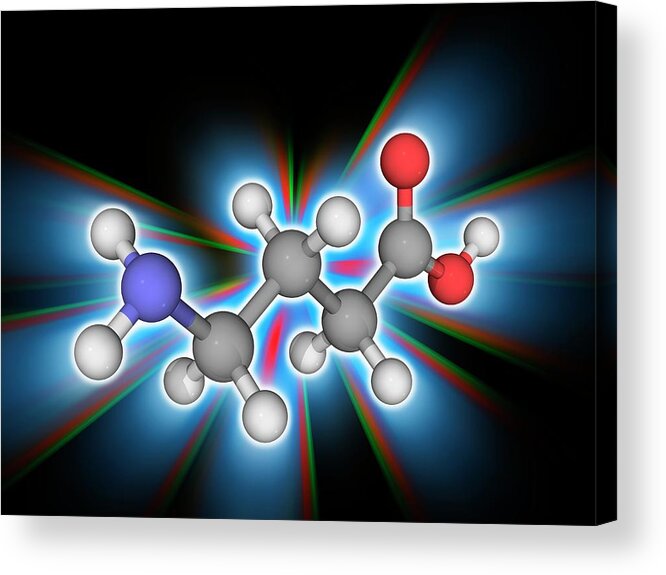This vibrant digital poster features a detailed and artistic depiction of a molecule chain. The primary structure includes one main blue circle, four main gray circles, and smaller connecting circles in white and red. The blue circle is accompanied by two small white circles, while the gray circles each have connections, with the fourth gray circle attaching to two small red circles, one of which also has a small white circle.

The background is dynamic, transitioning from dark to light blue with an overarching black backdrop. This is interwoven with striking starburst rays in red, green, and blue, adding depth and a glowing effect. This composition, devoid of text, combines scientific accuracy with bold, eye-catching colors, evoking the intricate beauty of molecular structures.